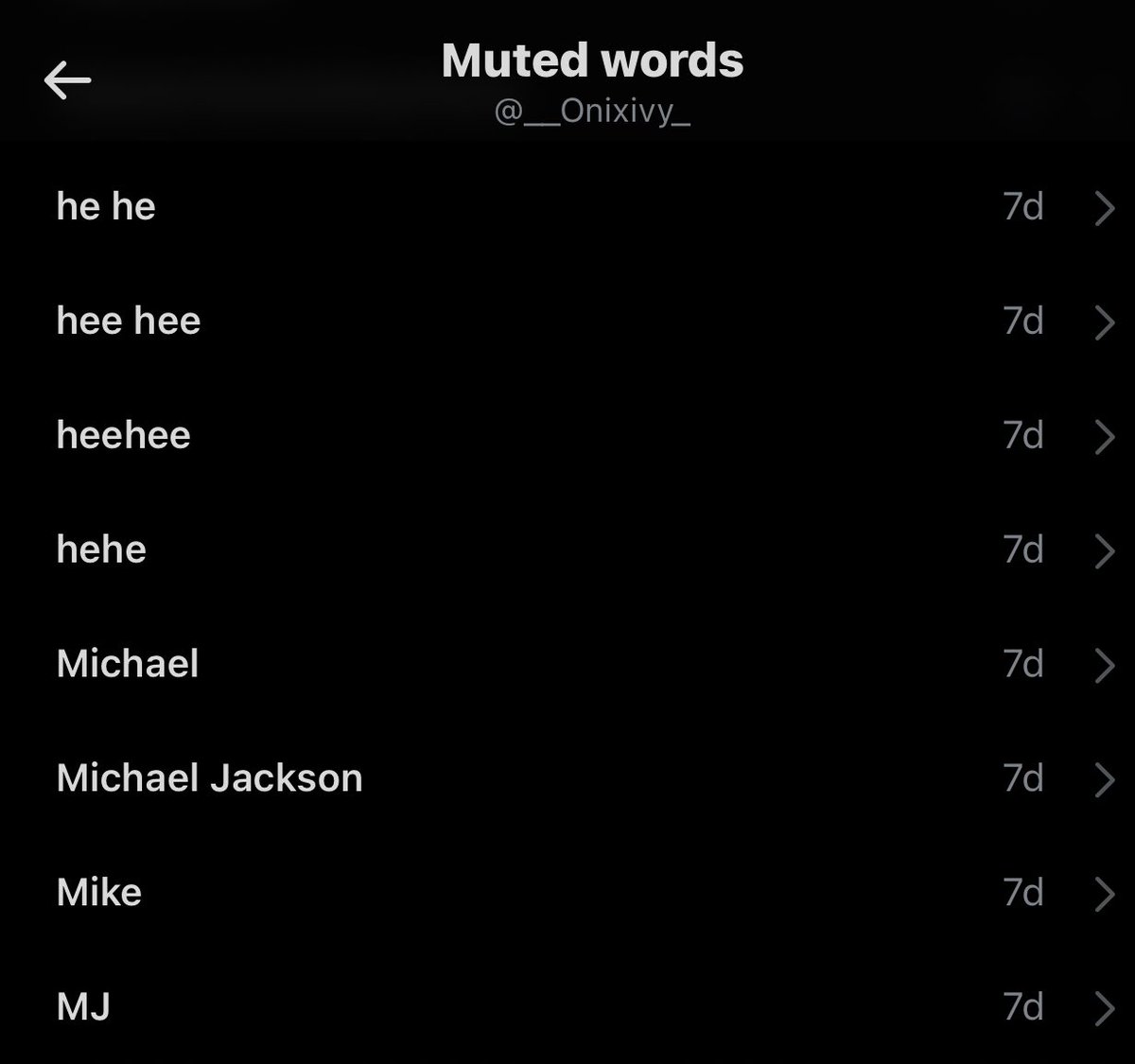Screenshot of a webpage or application displaying a user's muted words list. The header at the top is black, featuring white and gray text with a back arrow on the left reading “@Onyxiv_”. The content appears to be a vertical list of words or phrases marked as muted, each followed by the duration “seven days” indicated by a forward arrow symbol:

1. "he, he, seven days"
2. "he, he, seven days"
3. "he, he, seven days"
4. "he he, seven days"
5. "Michael, seven days"
6. "Michael Jackson, seven days"
7. "Mike, seven days"
8. "MJ, seven days"

This list suggests that the user has temporarily muted various spellings and iterations of certain terms, primarily related to "he, he" and different forms of the name Michael or MJ, for a duration of seven days each.